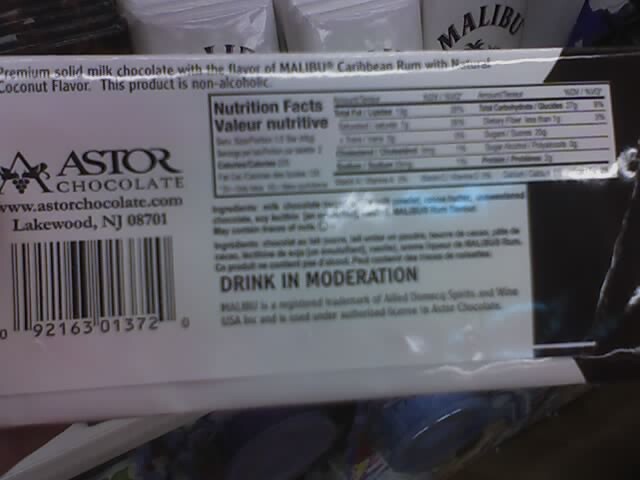The photograph, which is wider than it is tall, captures an assortment of chocolate brands in a store setting. The focal point of the image is a bar of Astor premium solid milk chocolate, flavored with Malibu Caribbean rum, held by a person who positions the nutritional facts towards the viewer at the bottom of the image. This Astor chocolate originates from Lakewood, New Jersey, 08701. 

Although the nutritional information is somewhat blurry, it indicates that the chocolate contains approximately 7-8% of the daily intake of carbohydrates or glucose, along with 2% dietary fiber, and around 30% of the daily intake of total fat. At the very bottom of the package, the phrase "drink in moderation" is visible. 

In the background, further away from the chocolate bar being highlighted, various other chocolate brands are displayed, with the front packaging of some chocolates, including another Malibu Rum Chocolate, discernible among the assortment.